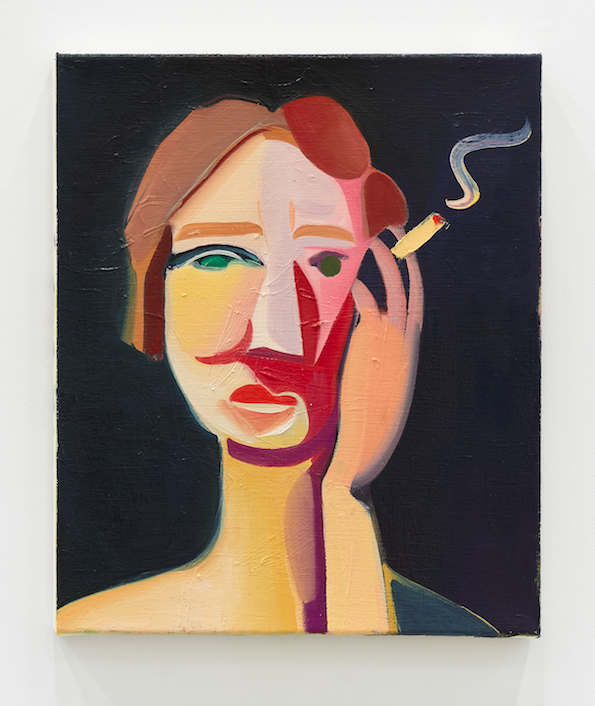This vertically aligned rectangular painting, reminiscent of Picasso's cubist style, features a figure—possibly a woman—smoking a cigarette. The figure has short brown hair that slightly covers the ears, and green eyes, with one eye significantly larger than the other. The facial features are highly exaggerated and distorted, using large brushstrokes to create a jarring, impressionistic effect. 

The face displays a stark contrast in makeup; one side is adorned while the other remains bare. The complexion varies with areas of beige, tan, and pink, and there's a distinct purple line running down the chin and neck. Adding to the asymmetry, the nose appears as an abstract collection of brushstrokes rather than a defined shape. The upper lip is brown, the lower lip tan, and the eyelids are marked with black. One shoulder is gray, while the other is a beige-yellow hue. 

The left hand is raised to the side of the head, as if holding a phone, and grips a yellow cigarette with a red interior, from which smoke billows upward. The image is set against a textured black background, framed by a light gray border, and hangs on a white wall. No artist's signature is visible on the canvas.